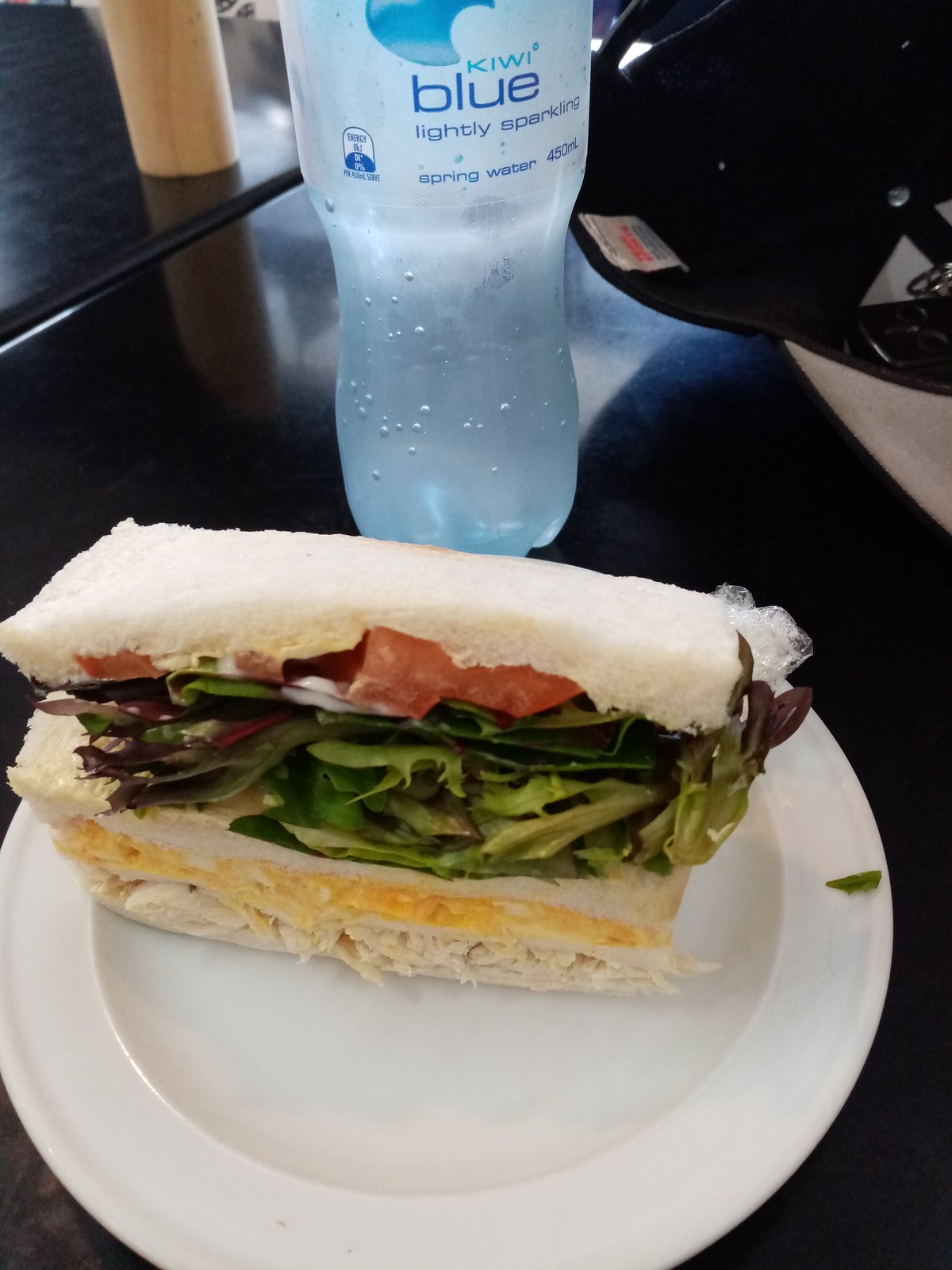A close-up photograph features half of a meticulously layered sandwich resting on a pristine white plate, placed on a dark, textured table. The sandwich is crafted with three slices of soft white bread. The base layer showcases either succulent turkey or tuna, topped with a slice of creamy cheese. Above this, the middle slice of bread provides a stable structure for the fresh, leafy lettuce and vibrant red tomato slices that crown the creation, finishing with the top layer of bread. In the background, a bottle of sparkling water stands tall, its surface glistening with beads of condensation, suggesting it has just been retrieved from a cold environment.